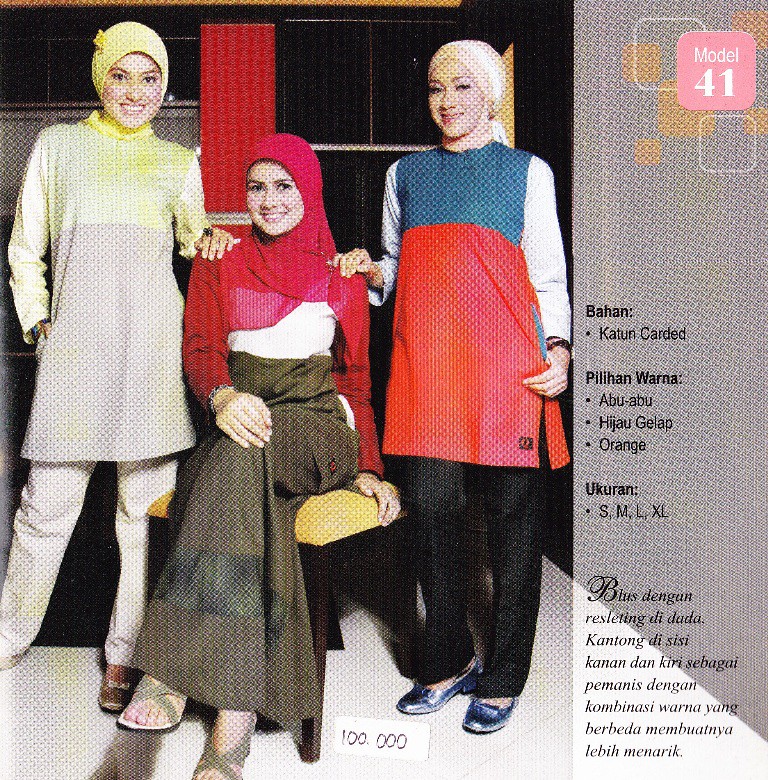The photograph features three women, each adorned with intricate headscarves that cover their hair but leave their faces visible. The central woman, seated on a yellow seat labeled "Model 41," wears a red shawl over a brown dress. To her left, a woman stands in a gray outfit with yellow accents and a matching yellow headdress. On the right, the third woman sports a red, blue, and white top paired with black jeans, blue shoes, and a white and tan headdress. All three women smile warmly, with the standing women resting their hands on the seated woman's shoulders, symbolizing a sense of camaraderie. The image also contains text in an unfamiliar language that includes descriptions of the outfits and size options, suggesting it might be part of an advertisement targeting potential buyers of these traditional gowns. The background features a pink box with white font stating "Model 41," and additional details are written in black and orange fonts.